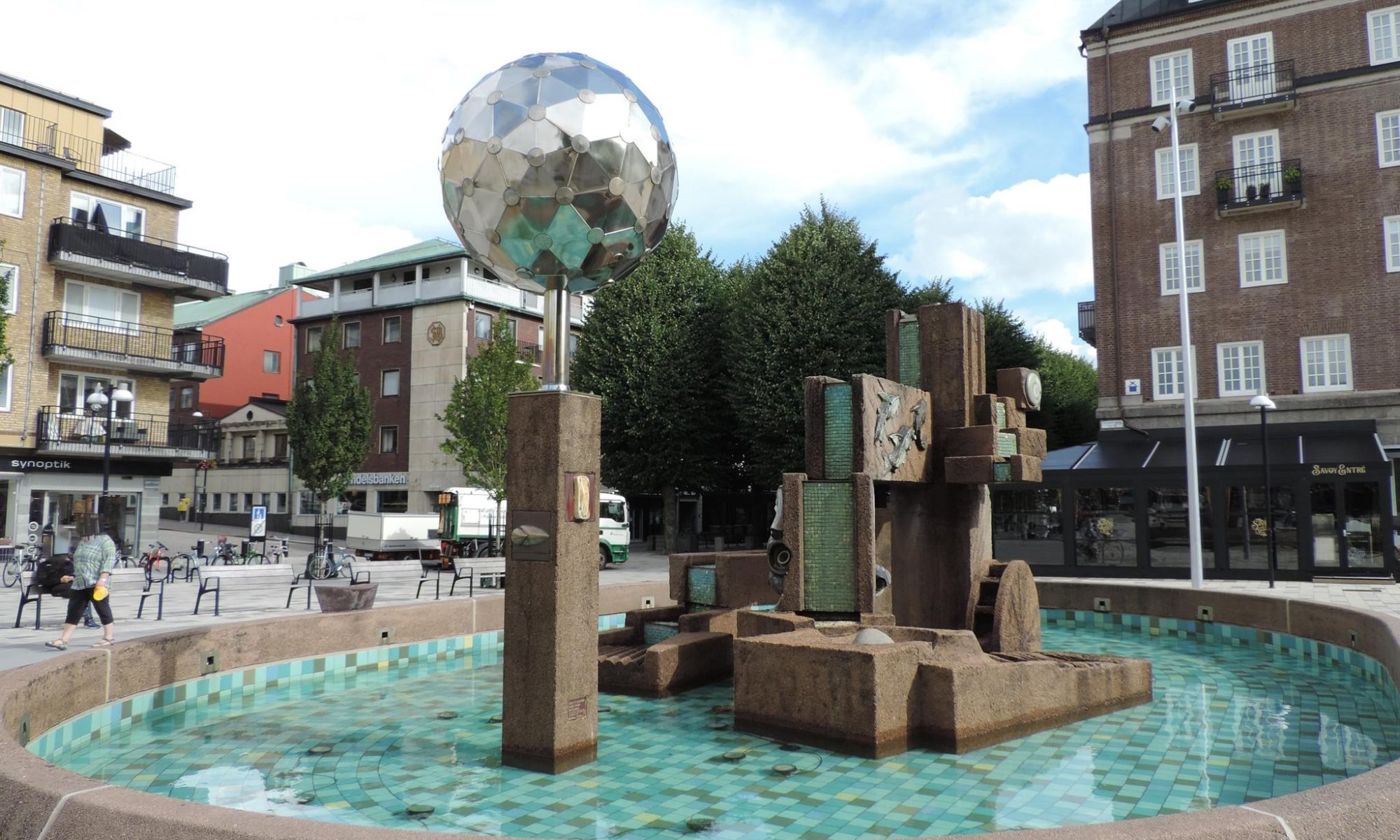The image captures a modern art installation in the center of a town square pool. The focal point is a tall, brownstone column topped with a large, silver disco ball adorned with geometric dot patterns. Surrounding this column are an array of stone decorations, including stacked stone formations reminiscent of Jenga blocks. The pool, circular in shape, is lined with a mosaic of small tiles in varying shades of green, blue, black, gold, and brown, though it appears to be holding a low level of water. To the left, parked bicycles and a person walking can be seen. In the background, apartment buildings—one brown with white windows and black balconies, another reddish—frame the scene against a light blue sky laced with white clouds. The rim of the pool is made from light brown stone, enhancing the overall composition of the image.